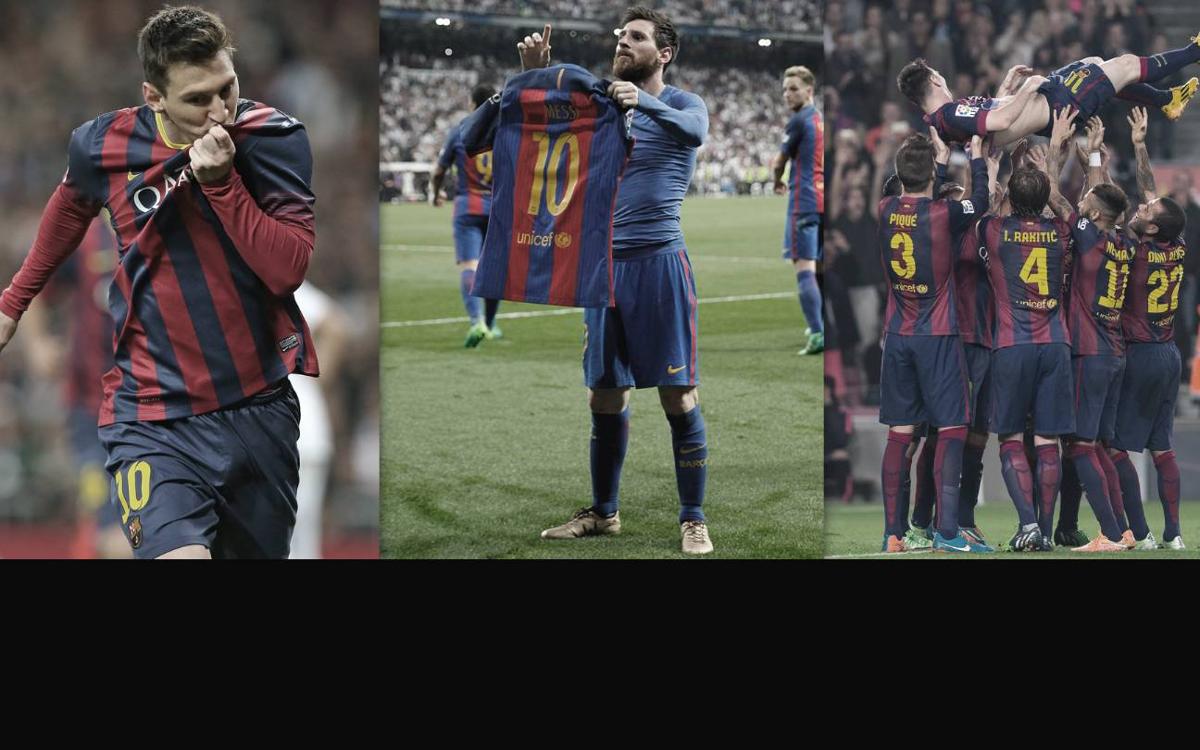The image is a 6-inch wide by 3-inch high rectangular collage consisting of three equal-sized photographs on the top two-thirds, with the bottom third being a plain black footer. The first photo on the left depicts a Caucasian athlete on a soccer field. He has short brown hair and is wearing a red and black vertical-striped jersey with solid red sleeves and a yellow collar. The athlete is also wearing black shorts with a gold number 10 on them. He is pulling up his shirt to wipe his mouth, obscuring the white print on the front of the shirt. The background behind him is blurred. In the middle photo, another man of Caucasian descent, with brown hair and a mustache and beard, stands in front of a crowded stadium. He is dressed in a tight-fitting, long-sleeved blue shirt with matching blue or black shorts that include a gold Nike symbol and a red stripe down the side. He also wears blue or black knee-high socks with some kind of gold design. His left arm is raised and bent at the elbow, holding up a jersey that reads "Messi," with the number 10 and "UNICEF" in gold. His right arm is extended with his index finger pointing up. The final photo on the right shows a group of athletes hoisting another player into the air on their hands. They are all wearing matching red and navy blue or black jerseys with black shorts and knee-high socks. Visible numbers in gold include 3, 4, 11, and 27, with some of the named players being Pique (3) and Rakitic (4). The central figure being lifted appears to be enjoying the moment, suggesting a celebratory scene, possibly related to a retirement ceremony.